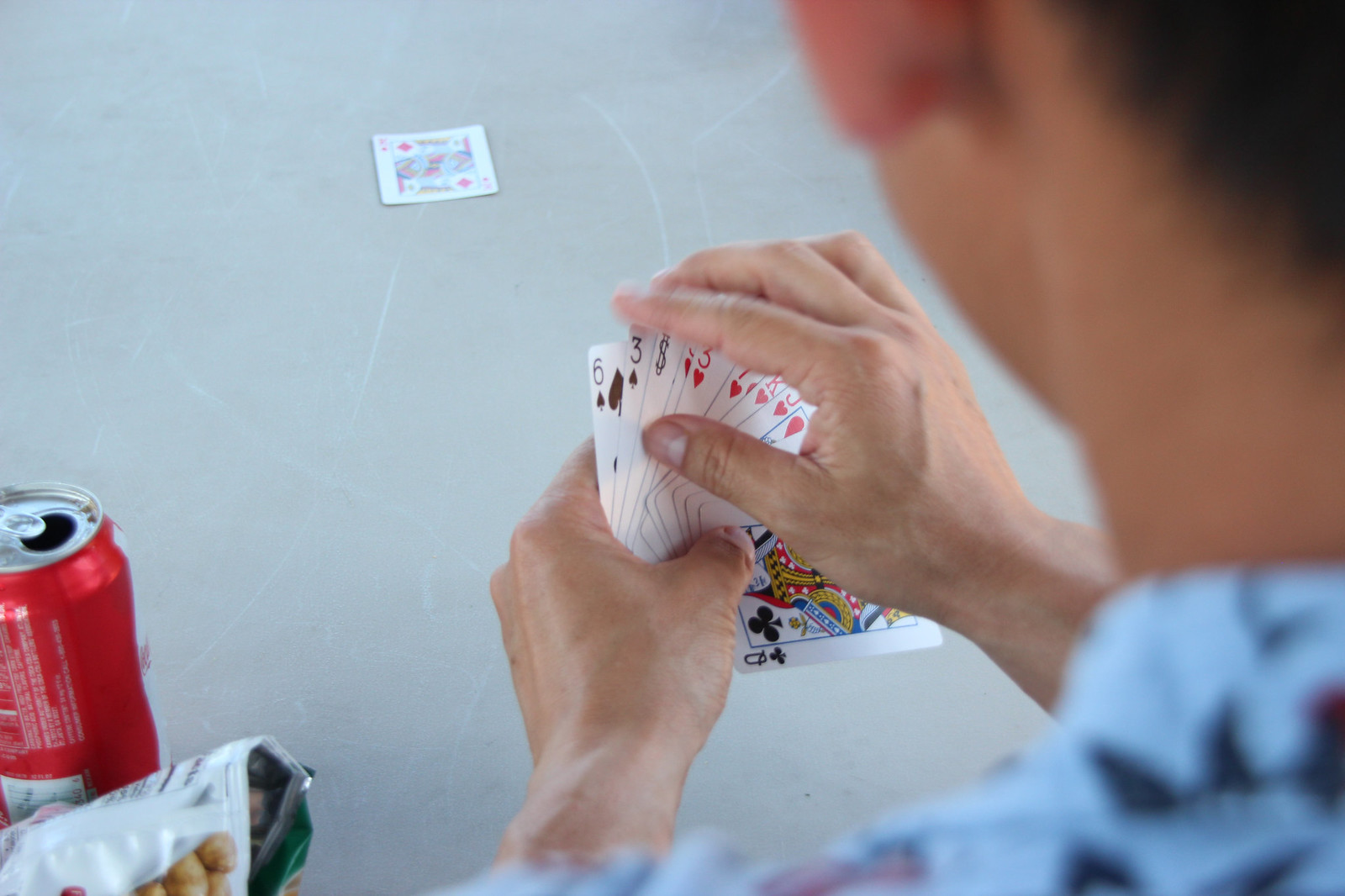In the image, a person, likely a man based on the blurred view of the back of their neck and ear, is seen from behind, holding a fan of nine playing cards in both hands. The cards are partially obscured by his right hand, but visible cards include a 6 and a 3 of spades, a Joker, a 3, 7, King, and Jack of hearts, and a Queen of clubs. In front of him is a scratched, white table with a single King of diamonds card face-up in the distance. To the left of the person sits an open red can of soda, likely Coca-Cola, and an open bag of potato chips just in front of the soda can.